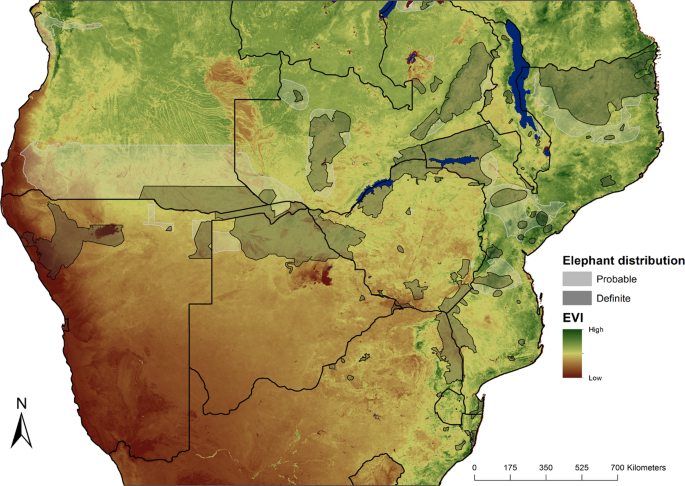This is a detailed close-up map of central Africa, highlighting elephant distribution and the Enhanced Vegetation Index (EVI). The map displays countries outlined in black with various topographic colors—green, brown, orange, and gray. The green areas indicate high EVI, moving to yellow, light green, gold, light gold, orange, and red for lower EVI values. The key on the right explains the elephant distribution: light gray areas indicate probable elephant habitats, while dark gray areas indicate definite habitats. Prominent lakes and rivers are colored blue. To the right, the text "Elephant Distribution" is noted in black. The bottom features a mileage line indicating distances up to 700 kilometers, and an arrow pointing north on the left side.